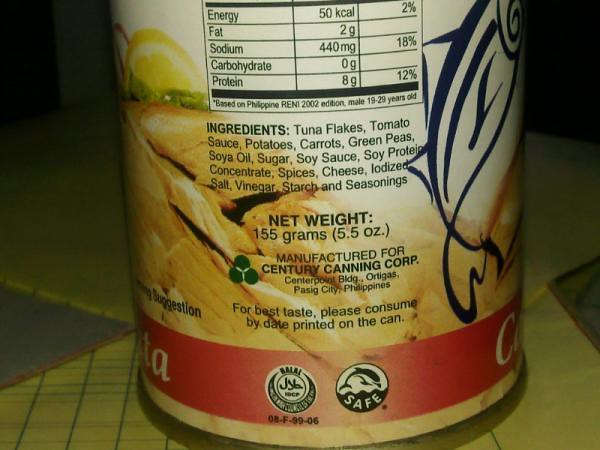The image showcases a tall tin can with a detailed label, most likely containing a tuna-based product. The label prominently features a tuna logo, indicating the main ingredient. The bottom section includes the nutrition facts and a detailed list of ingredients: tuna flakes, tomato sauce, potatoes, carrots, green peas, soy oil, sugar, soy sauce, soy protein, concentrated spices, cheese, iodized salt, vinegar, starch, and seasonings. The product, manufactured by Century Canning Corporation in High Seas City, Philippines, is encased in a standard cylindrical tin can.